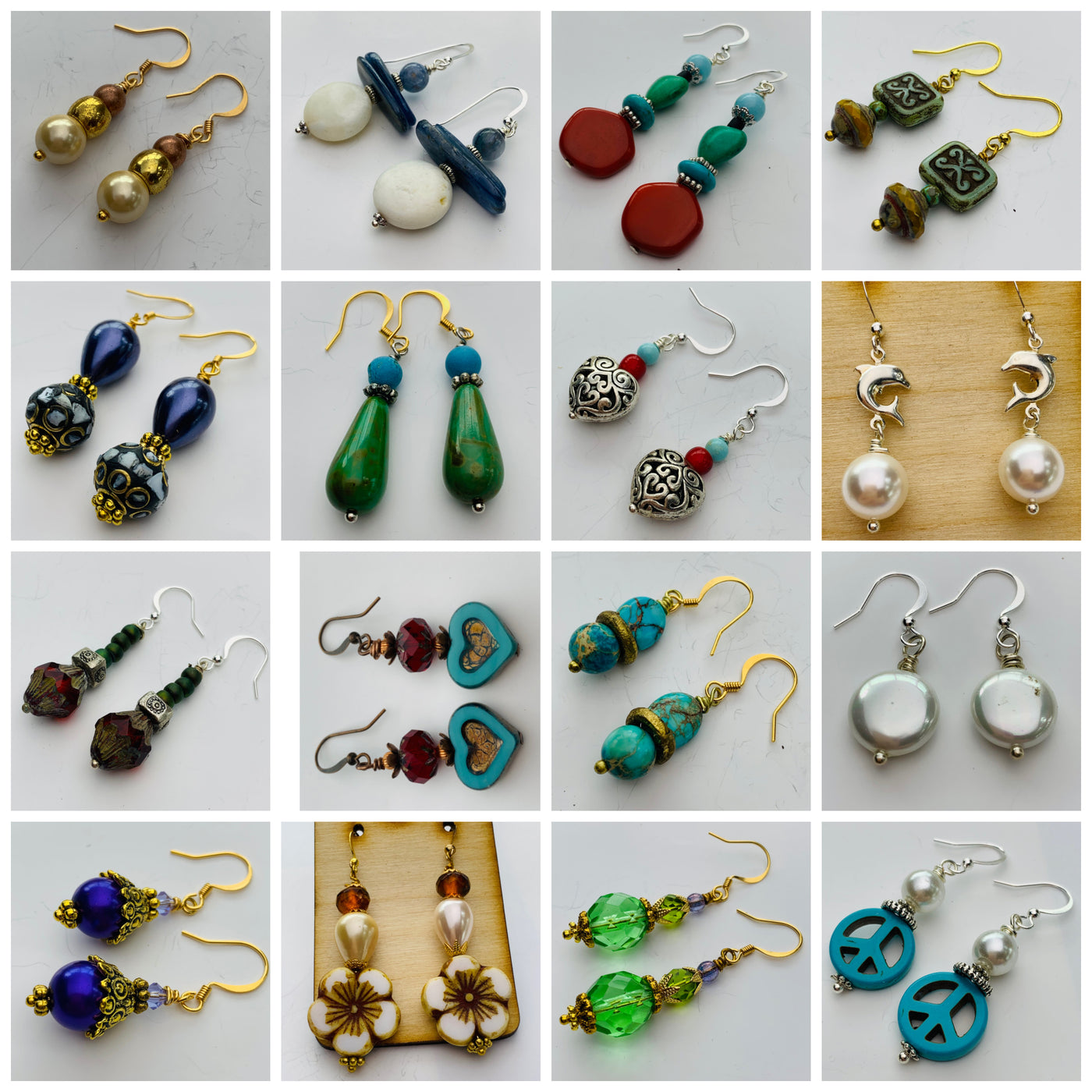The image showcases an assortment of 16 distinct pairs of earrings, each displayed within its own square on a white grid, forming a 4x4 layout. Each pair is unique in design, color, and shape, reflecting a wide variety of styles and materials. The top left earring features a golden design with three cylindrical beads in descending colors of brown, gold, and white. The bottom right showcases a turquoise peace symbol with a pearl atop, which stands out as particularly notable. Among these are earrings with golden pearlescence, moon and flying saucer shapes, clay-like beads in red, green, and blue, and intricate South American-inspired patterns. Some earrings display blue beading with green teardrops, antique pewter hearts with detailed designs, and pearls topped with silver dolphins. There are chunkier designs resembling natural stars, blue hearts with beadwork, turquoise beads separated by golden rings, as well as ornate pairs with purple and royal blue accented by gold filigree. Additionally, two pairs resemble atomic glass with green gemstone cuts and creamy floral designs with red beads. Each pair is matched within its respective square but distinct from the others, offering a rich and varied collection of earring styles.